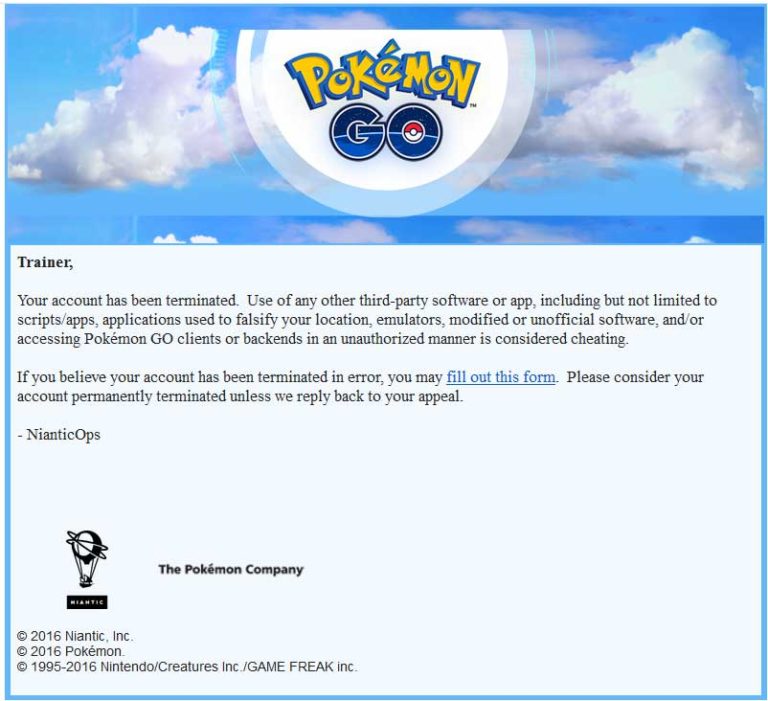The image features a notification message from Pokémon GO, set against a backdrop with a blue sky at the top. The Pokémon GO logo is prominently displayed, accentuating the subject of the message. The text in the notification reads:

"Trainer, your account has been terminated due to the use of unauthorized third-party software, including but not limited to scripts, apps, applications used to falsify your location, emulators, modified or unofficial software, and unauthorized access to Pokémon GO clients or backends. This is considered cheating. If you believe your account was terminated in error, you may fill out the provided form. Please consider your account permanently terminated unless we respond to your appeal."

The message is attributed to Niantic Ops and bears the logos of Niantic and The Pokémon Company, with a copyright notice indicating the year 2016.